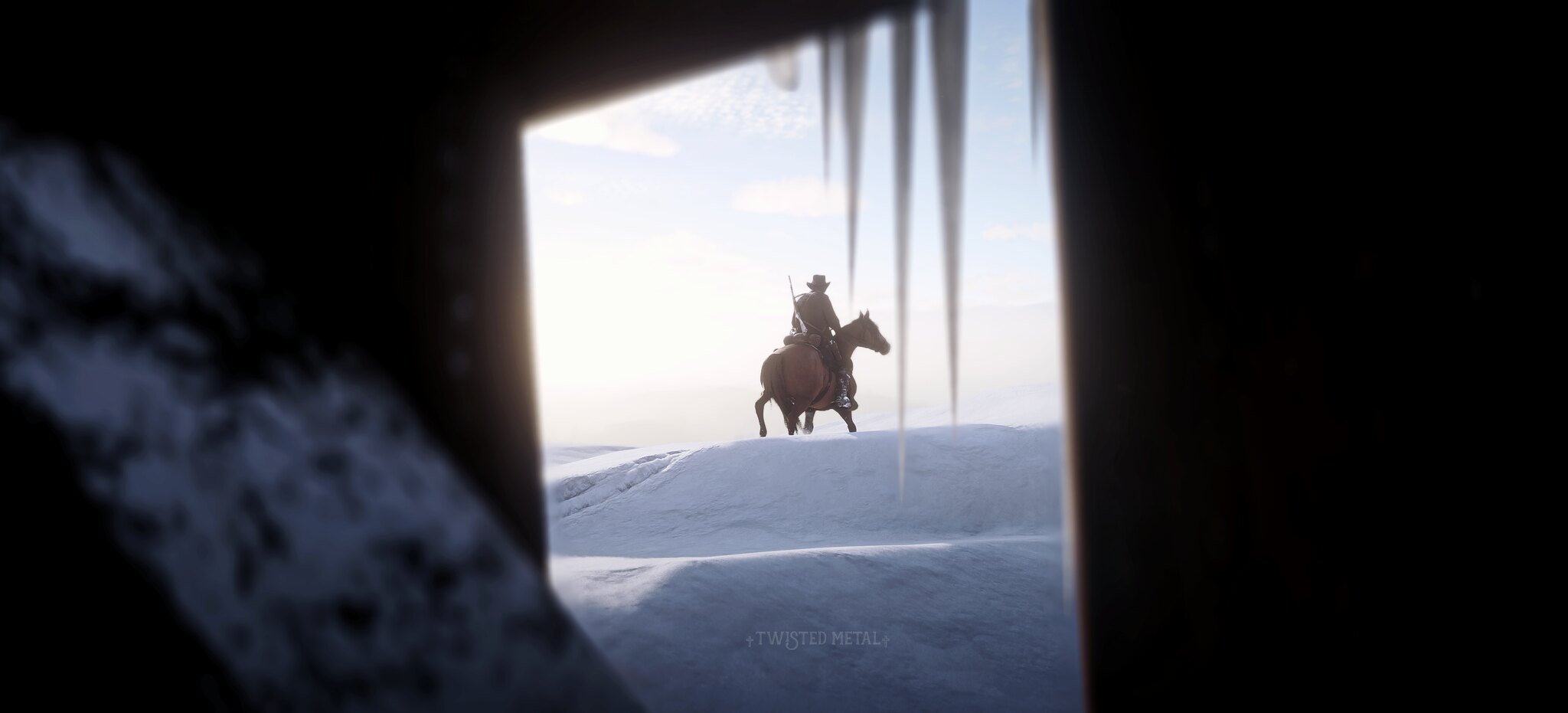This detailed screenshot from the video game Red Dead Redemption 2 captures an evocative scene centered around a lone cowboy. Sitting astride a brown horse, the cowboy is positioned in the distance at the center of the image, standing resolutely atop a snow-capped hill with two distinct levels, occupying the highest point. The cowboy, identifiable by his wide-brimmed hat and long gun strapped across his back, is framed perfectly by a rectangular door frame. This door frame, weathered and brown, suggests that the image is taken from within an abandoned house, adding to the atmospheric charm of the scene. To the right of the doorway, icicles dangle menacingly from the top of the image, hinting at the harsh winter conditions. An additional detail includes a snow-laden plank of old wood, positioned diagonally from the top left corner and slightly obscuring part of the doorway, further emphasizing the dilapidated state of the shelter. This captivating image conjures a sense of solitude and resilience in the face of a rugged and unforgiving landscape.